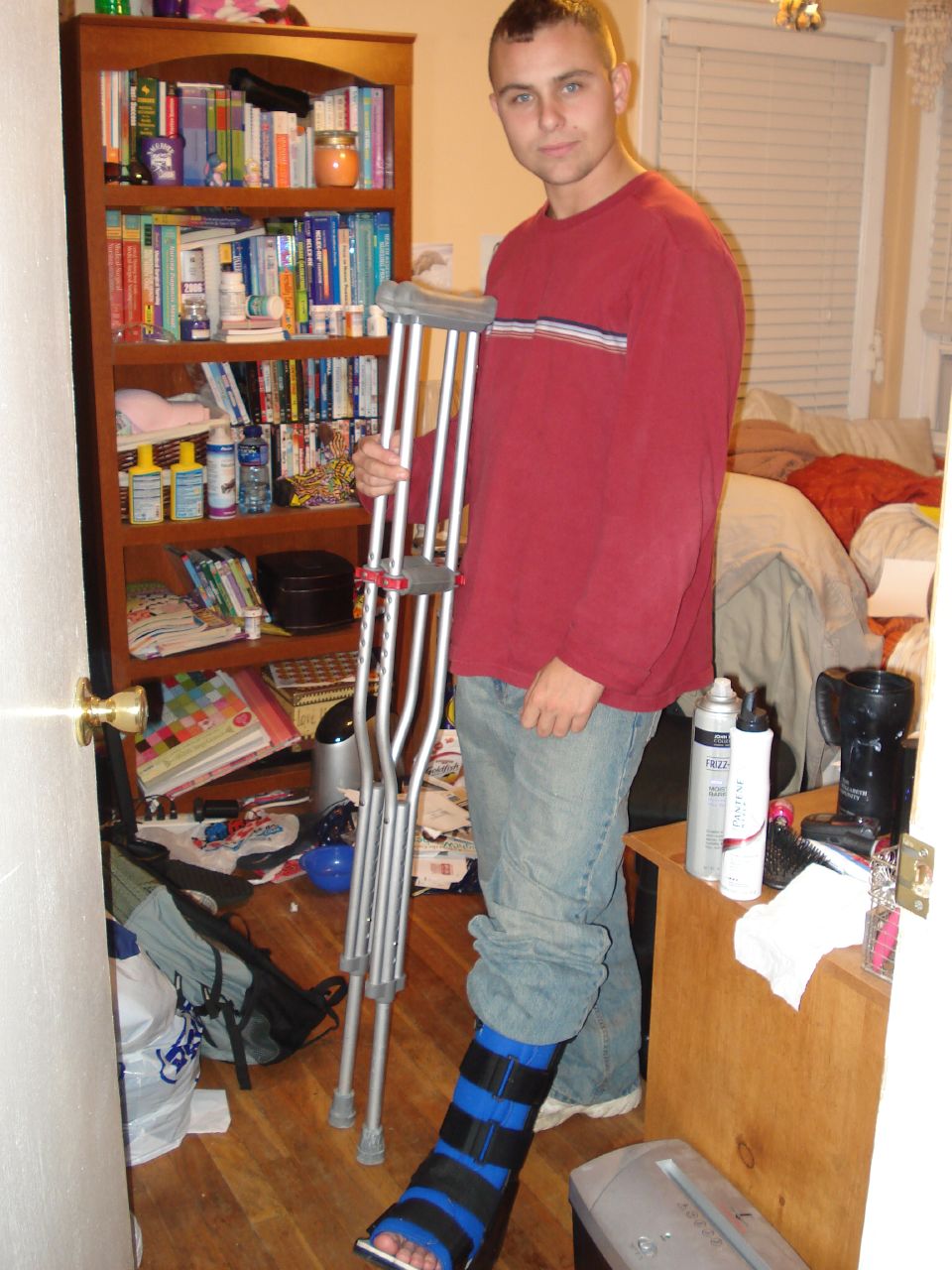This is a detailed photograph capturing a young man with short brown hair and blue eyes standing in a cluttered, yellow-walled room with a brown wooden floor. The man is holding a pair of silver crutches with a touch of red on the handles in his right hand. He is wearing blue jeans and a long-sleeve red sweater adorned with blue, light blue, white, and pink bands in the center. His left foot is encased in a blue cast wrapped with black belts, while a white shoe covers his non-casted right foot. 

To his left, there is a wooden bookshelf brimming with various colorful books and numerous bottles, including what appears to be a prescription bottle and a large black container on the second shelf from the bottom. The bottom shelf holds large books and a yellow box with brown details. On a stand in the lower right corner of the room, positioned above a paper shredder, are more bottles that resemble shampoo containers, although their labels are illegible. Nearby, a drinking cup is also visible. 

In the background, behind and to the right of the man, there appears to be a haphazard pile of ten pillows, possibly on a bed. Among these pillows, there is a red sheet and a white pillow with some yellow. Additionally, there are two windows; one directly behind him has closed blinds, while the other, to the right, has its blinds slightly open. The room's scattered debris includes what seems to be a backpack, adding to the overall cluttered appearance.